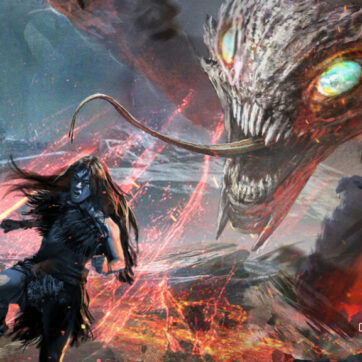The image depicts a detailed close-up of a menacing extraterrestrial reptilian creature's face. Its skin is a mottled gray, and it possesses striking, piercing blue eyes. The creature's mouth is open, revealing sharp, jagged teeth and a long, extended tongue, as if it is poised to capture something. The background is a surreal and hazy blend of red, green, and black hues, enhancing the otherworldly ambiance. The central focus remains on the monstrous creature, highlighting its sinister and predatory features against the eerie backdrop.